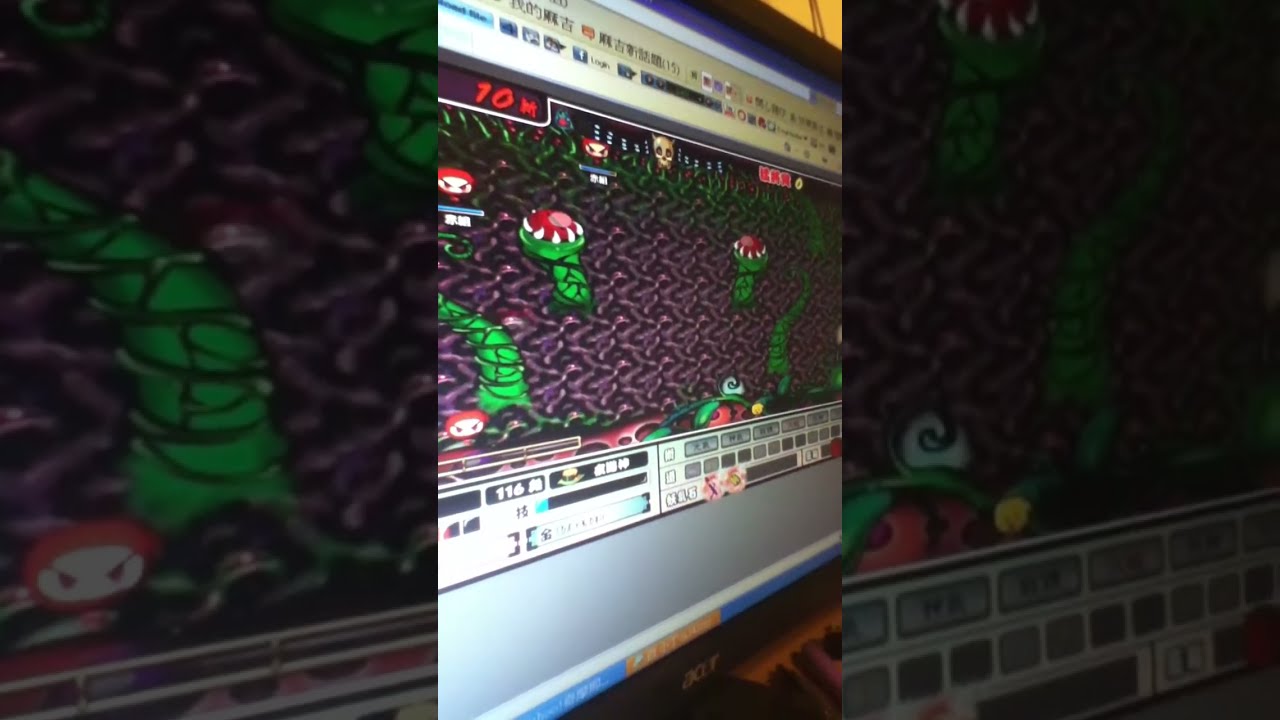In this image, the primary focus is an Acer computer monitor positioned centrally, taking up most of the middle panel of a three-panel layout. The left and right panels of the image are entirely black, providing contrast to the brightly lit middle panel. The monitor displays a Windows Internet Explorer browser tab at a skewed 45-degree angle, giving a partial view of the screen. On the screen, we see a computer game featuring a fantasy setting with various visual elements: plants with teeth emerging from the ground, red circular creatures with white faces and large red eyes, and additional colorful graphics. The game interface includes multiple toolbars and taskbars, filled with game-related information such as bar graphs and health bars, all adorned with text in a foreign language, likely Chinese. The scene appears to be in an indoor gaming room, depicting a vibrant array of colors including blue, white, black, red, light blue, gray, green, pink, and purple.